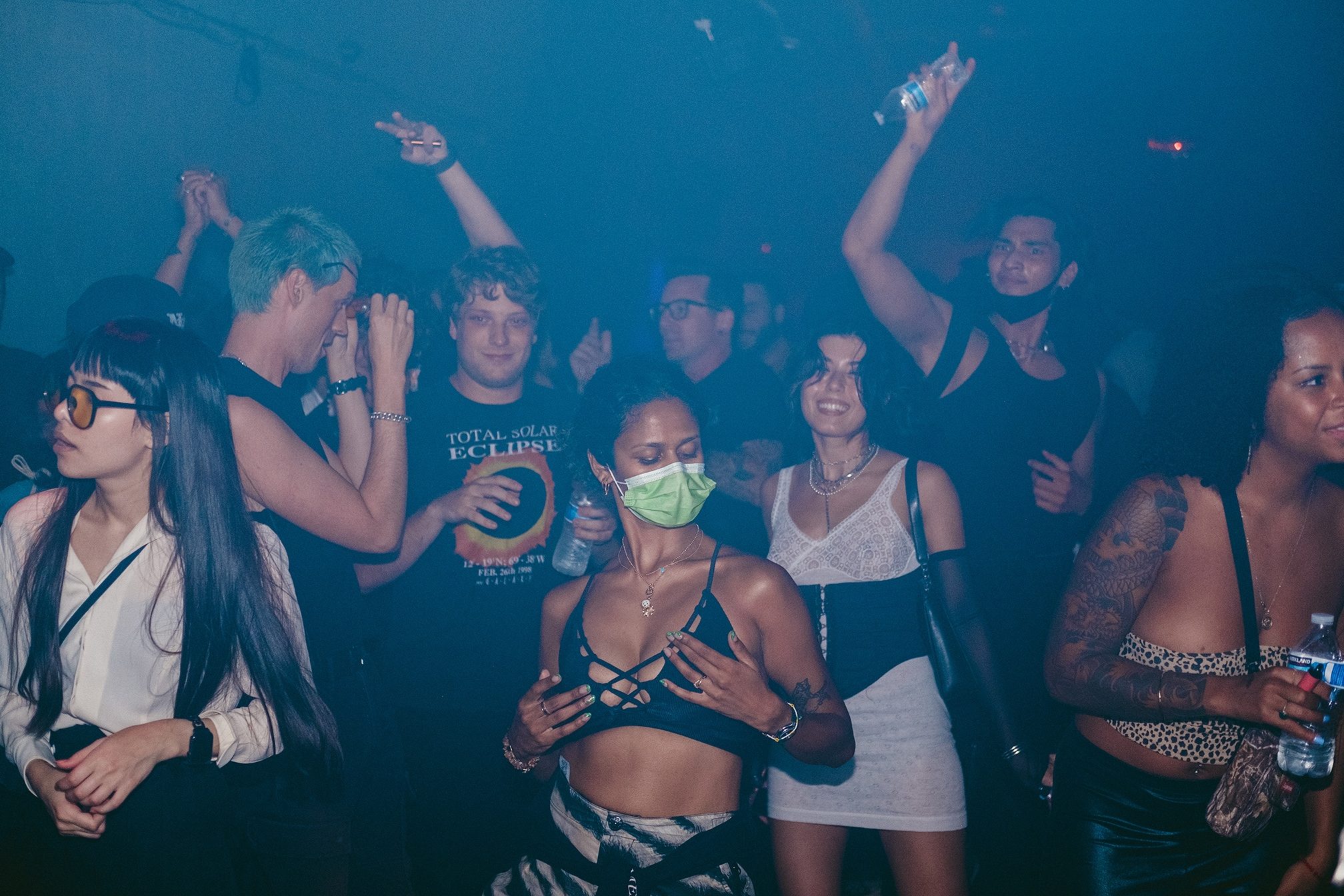The color photograph captures the lively atmosphere of a party at an eclipse event, likely set in a nightclub with a blue-hued, foggy room and white background walls. In the foreground, a woman with a green and white mask and a black sword bra outfit holds her breasts while dancing in black and white striped pants. To the right, a woman with long black hair dons a white lace dress with a black corset, black high sleeves, and a black purse. Nearby, a short man with blue hair, dressed in black clothing and jewelry on both wrists, stands out. Next to him, a man in a black Total Eclipse t-shirt with curly brown hair raises his hand. Another man, wearing a mask around his chin and a black daigo-tee, also raises his hand, gripping a water bottle with a blue label. A woman in a cheetah tube top with tattoos along her arm holds a water bottle. Far left, a person in black-framed sunglasses with brown lenses, a white shirt, black pants, and a black watch looks rightward. Completing the scene, a woman in a long-sleeved shirt and sunglasses, and another in a black camo bag holding a water bottle add to the vibrant crowd enjoying the eclipse celebration.